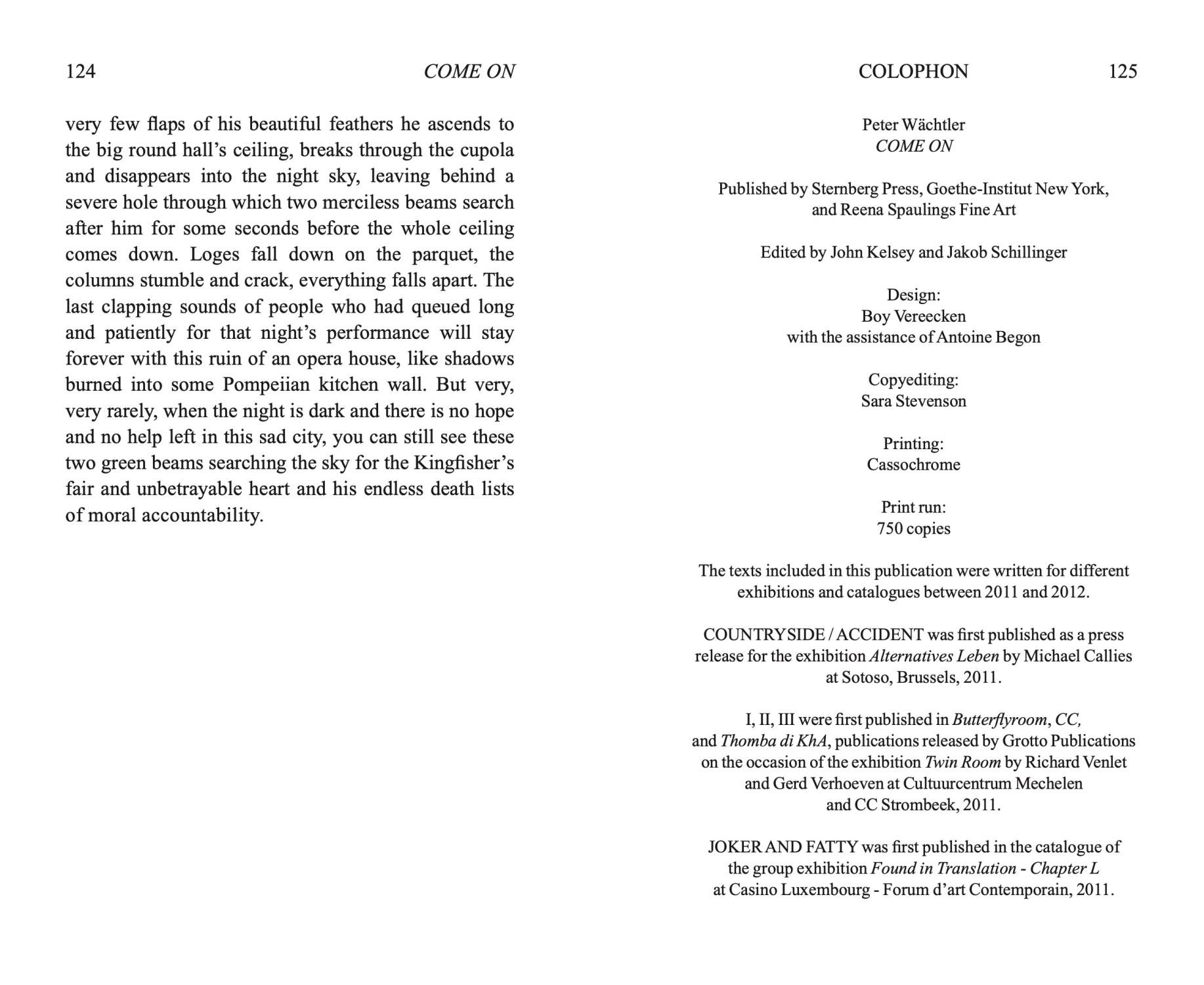The image shows a scanned spread from a book, displaying pages 124 and 125. On the left, page 124 features the concluding paragraph of a text, which includes a description involving "feathers and clapping sounds of people who had queued long and patiently for that night's performance." Above this paragraph, the title "Come On" is prominently displayed. Page 125, marked as "colophon," lists the publication details: "Come On" by Peter Wachtler, published by Sternberg Press in collaboration with the Goethe Institute New York. The editorial team includes Reena Spaulding for fine art editing and John Kelsey and Jacob Schillinger as editors. The design was led by Verican with assistance from Antoine Vigon, and copy editing by Sarah Stevenson. Coastal Chrome handled the printing, with a print run of 750 copies. This page represents the final credits and acknowledgments of the book.